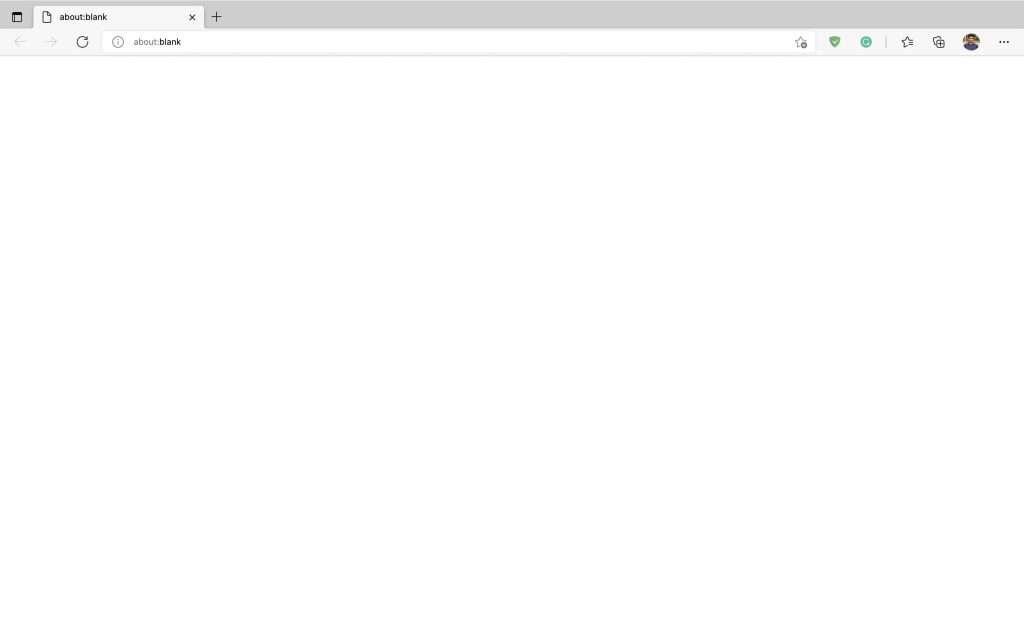The screenshot captures a web browser interface with intricate details. At the very top, there is a solid gray banner stretching horizontally across the screen. On the left side of the banner, a small square is partially darkened in black at the top. Below this, just slightly inward from the edge, runs a vertical line.

Moving rightward, there is an open browser tab, symbolized by a small paper icon with a folded top-right corner. This tab displays the text "about:blank" in lowercase letters, indicating the address of the open page. Adjacent to the right side of the tab label is an 'X,' used for closing the tab. Further to the right, on a darker gray background, sits a plus sign for opening a new tab.

Beneath the tab row, another section shows navigation controls including a left arrow, right arrow, and a refresh button. The left and right arrows are grayed out, indicating they are currently disabled. The browser's address bar lies next in line, showcasing a light gray 'i' icon inside a circle on the left side, followed by the text "about:blank" where 'about:' is in a lighter gray and 'blank' is in black text.

To the right of the address bar, there are several icons: a star for bookmarking, a screen shield with a white check mark indicating security or an ad-block function, a bluish-green circular arrow symbolizing page reload, another star, a square with a plus sign possibly for adding to a reading list or similar function, and a circular user icon that may represent a profile or account option. Finally, three vertical dots complete the lineup, typically signifying additional options or a menu.